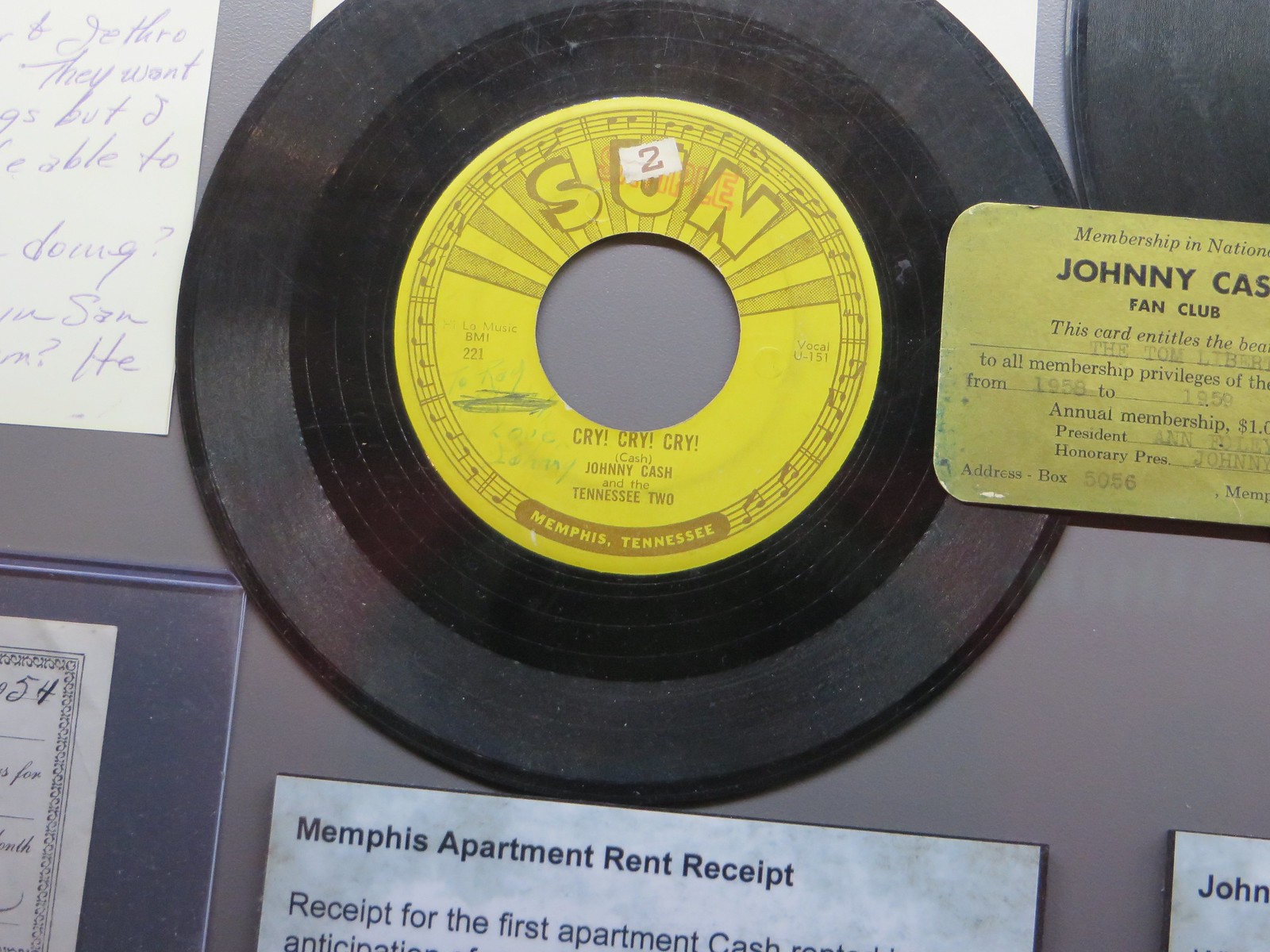The image is an indoor photograph dedicated to Johnny Cash, featuring a prominently displayed 45 RPM vinyl record at its center. The record, produced by Sun Records in the 1950s, has a large hole in the middle and bears the title "Cry, Cry, Cry" by Johnny Cash. To the right of the record, partially visible, is a Johnny Cash fan club card, which mentions membership entitlements. In the bottom section of the image, there is a cut-off placard that states "Memphis apartment rent receipt," indicating a receipt for Johnny Cash's first apartment, though the text is partly obscured. Additionally, in the upper left corner, there is a handwritten letter on a piece of white paper. The image features a color palette of black, yellow, white, blue, gray, and various shades of gray, suggesting it was taken in a music-related studio setting.